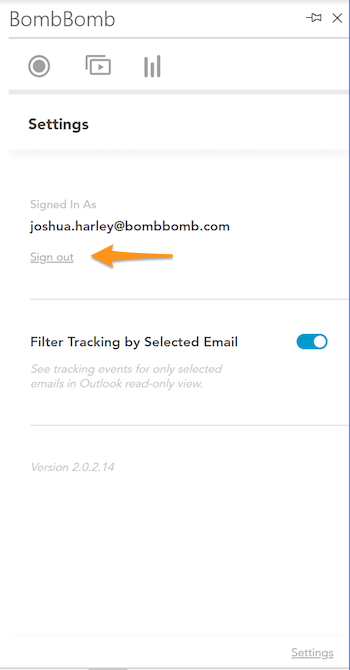This image depicts the settings page of an app or program, likely taken from a cell phone screen. The photo is in portrait orientation and features a narrow blue line running vertically along the right edge, creating a border. Horizontal gray lines frame the top and bottom, adding a subtle boundary.

At the top of the screen, the word "BombBomb" appears in black font accompanied by a pin icon and a forward arrow icon to the right. A slightly thicker gray line separates this header from the subsequent sections, which include a record button, a play button, and a graph button.

Below this, a thicker gray border is followed by the word "Settings" in black font, with another gray border beneath it. The subsequent section, in gray lettering, reads, "Signed in as Joshua.Harley at BombBomb.com," with a "Sign out" link directly below it. An orange arrow pointing to the left is placed adjacent to the sign-out link.

A thin gray divider then introduces the following section, which states, "Filter Tracking by Selected Email" next to a blue toggle switch in the "on" position. The description under this toggle explains, "See Tracking Events for Only Selected Emails in Outlook and Read Only View."

At the bottom, it notes the app version as "2.02.14" and includes a link to additional settings. While the precise function of BombBomb is unclear, this settings page appears to be configured for the user Joshua Harley's account.